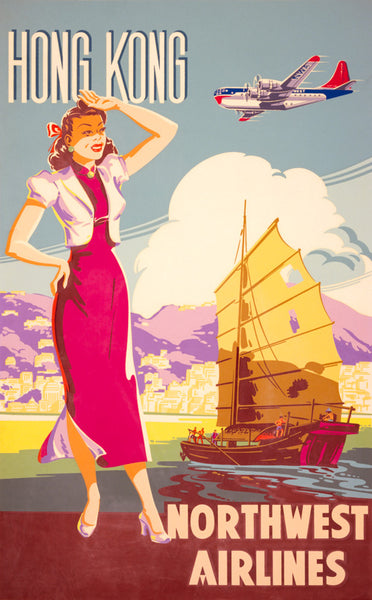This detailed lithograph-style poster advertises Northwest Airlines with a vibrant and nostalgic depiction of Hong Kong. The backdrop features a serene, blue sky dotted with clouds and purple-tinged mountains, indicating a picturesque horizon. Set against this is an urban scene with yellow-hued buildings suggesting a quaint village. Prominently in the foreground is a classic Asian wooden boat with a large, slightly tattered sail, painted in shades of brown and red, sailing on blue waters. To the left of the image, a woman dressed in mid-20th century fashion stands. She wears a calf-length red dress with a side slit and a short white jacket, and she's posed with her arm raised as if shading her eyes from the sun. Her outfit is accessorized with light purple pumps and a brooch. Above her, the words "Hong Kong" are emblazoned in white, capital letters, while an airplane soars above the boat to the right. The bottom of the poster prominently displays "Northwest Airlines," tying together the travel theme with a vintage allure through a palette of blues, pinks, purples, and yellows.